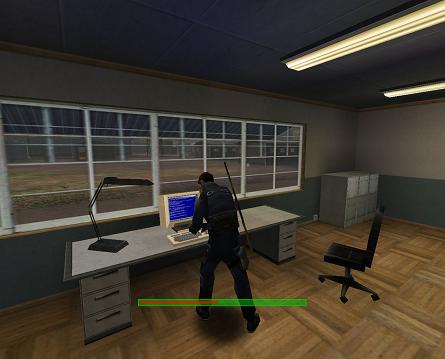This is a screen capture from a video game featuring a man in protective gear leaning over a computer at a sparse desk, which appears to be a desktop supported by two widely separated file cabinets. The man is typing on or hacking into the computer, indicated by the blue screen with white text reminiscent of an old-school text-based interface. The desk setup includes a minimalist black lamp, a computer with a beige monitor, and a black office chair pushed aside. The room resembles a general office space with a hard wooden floor and is sparsely detailed, characteristic of early 3D game graphics. In the background, there are three filing cabinets and three two-paned windows that offer a vague view of either a parking lot or some grass, possibly with buildings in the distance. The ceiling is equipped with two long fluorescent lamps. A green health meter at the bottom of the screen shows the character's health is half full, adding to the immersive gaming experience.